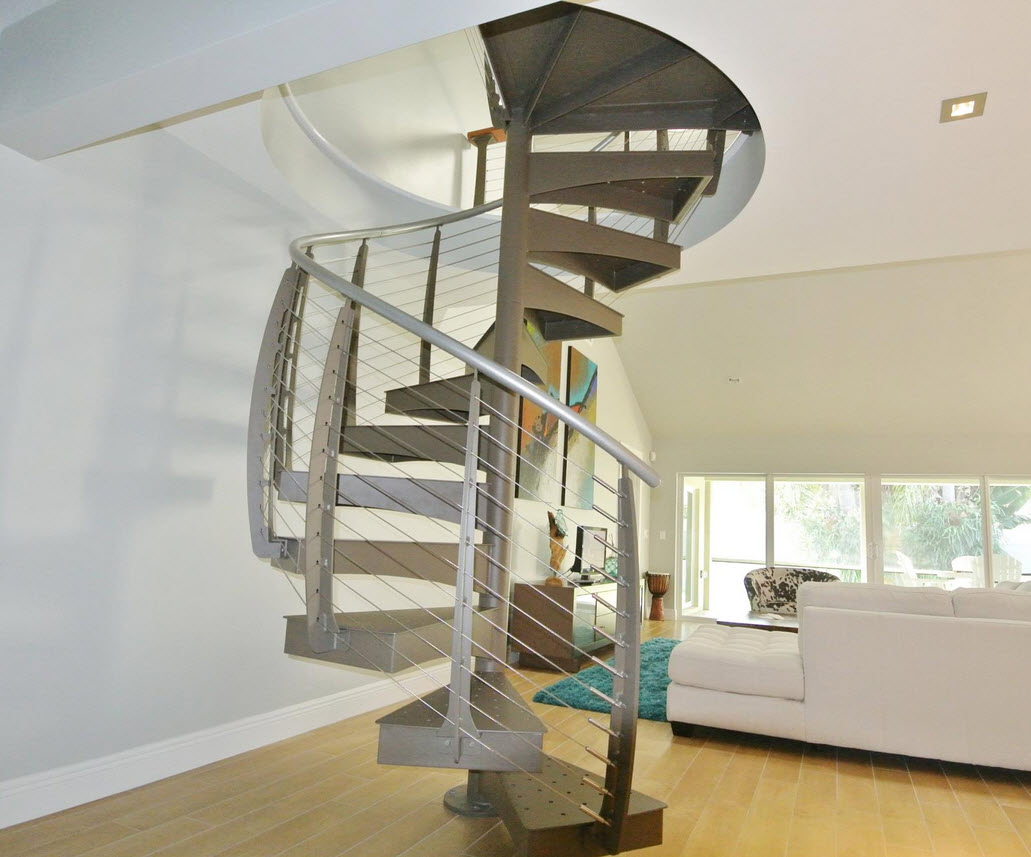The photograph captures a bright and modern living space with a distinct futuristic aesthetic. In the center of the room is a striking winding staircase featuring gray steps and a chrome handrail accentuated by thin metal wire safety bars. The walls are predominantly white, complementing the light brown wooden floors and contributing to the airy ambiance. 

On the right side of the room, a sleek white couch sits in front of a green rug, creating a vibrant contrast. Nearby, a TV rests atop a 3-foot stand, positioned against the wall. Large windows dominate the far right, allowing a flood of sunlight to illuminate the interior and offering views of lush greenery outside. 

Additionally, there's a small cabinet or stand adorned with a picture frame and possibly a statue, as well as some greenery. In the background, a sizable wicker basket adds a touch of rustic charm. The ceiling above the stairwell is also white, featuring a discreetly built-in light. Overall, the space combines modern elements with cozy touches, making it a visually appealing and inviting room.